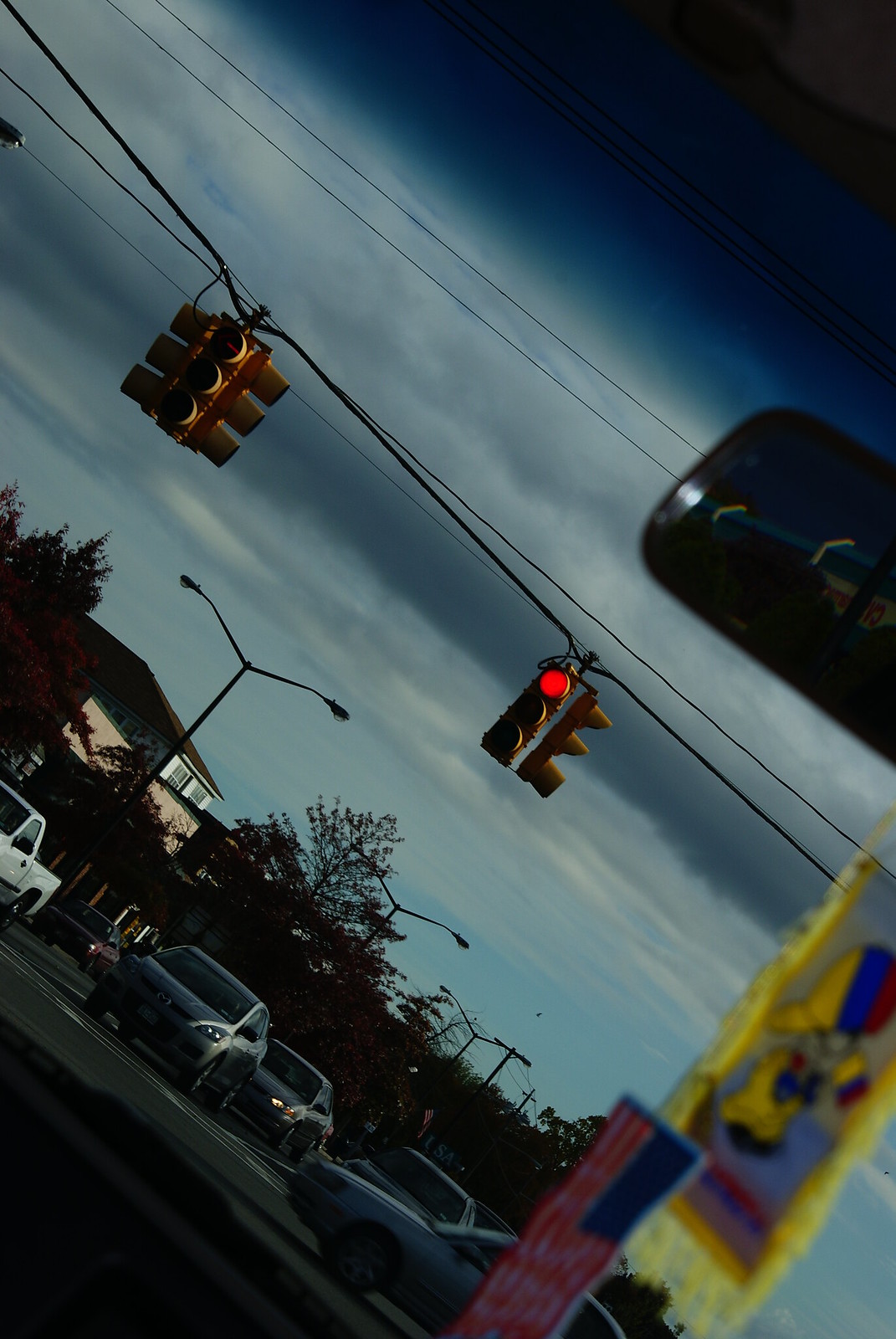The image depicts a scene at an intersection during an impending storm. The view from inside a car reveals a rearview mirror on the right side, adorned with a small American flag featuring red stripes and a blue section with stars at the top right, and another squarish piece of fabric with yellow edges and a blue center displaying an animated character. The sky above is an ominously dark blue, suggesting a storm is about to roll in, with white clouds below and electrical wires crossing the view. Hanging from one of these wires are two traffic lights; the one on the left is yellow and faces forward and to the sides, while the one nearer the center is red and operational, also facing forward and to the right.

Below, cars are positioned at the intersection, waiting at the red light, while other vehicles cross the intersection with the green light. Trees, houses, and inactive streetlights line the street in the background, with a few cars seen driving through the crossing.